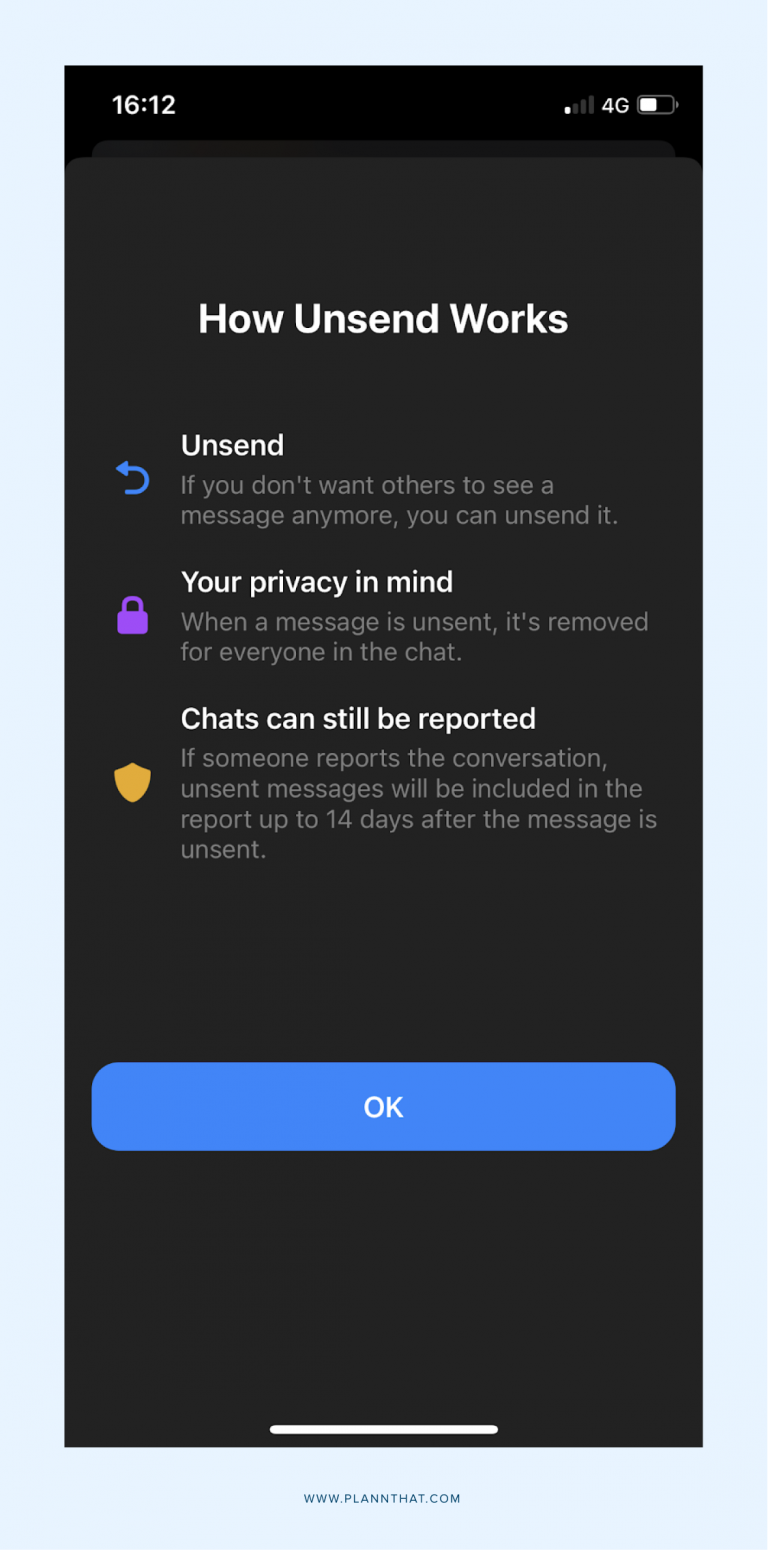The image features a light blue background, with a prominent black smartphone screen displayed at the forefront. The phone screen shows the time "16:12" and indicates a "4G" network connection. The main text on the screen explains the functionality of an "unsend" feature for messages.

At the top, the header reads "How Unsend Works," followed by a blue "Unsend" button. The detailed explanation states, "If you don’t want others to see a message anymore, you can unsend it." Below this is a purple lock icon accompanied by the message, "Your privacy and mine. When a message is unsent, it is removed for everyone in the chat."

Further down, a gold crest icon provides additional information: "Chats can still be reported. If someone reports the conversation, unsent messages will be included in the report up to 14 days after the message is unsent."

Towards the bottom of the screen, there is a large blue "Okay" button and a white stripe running along the bottom edge. Additionally, in the blue area near the bottom, the website "www.planthat.com" is displayed.